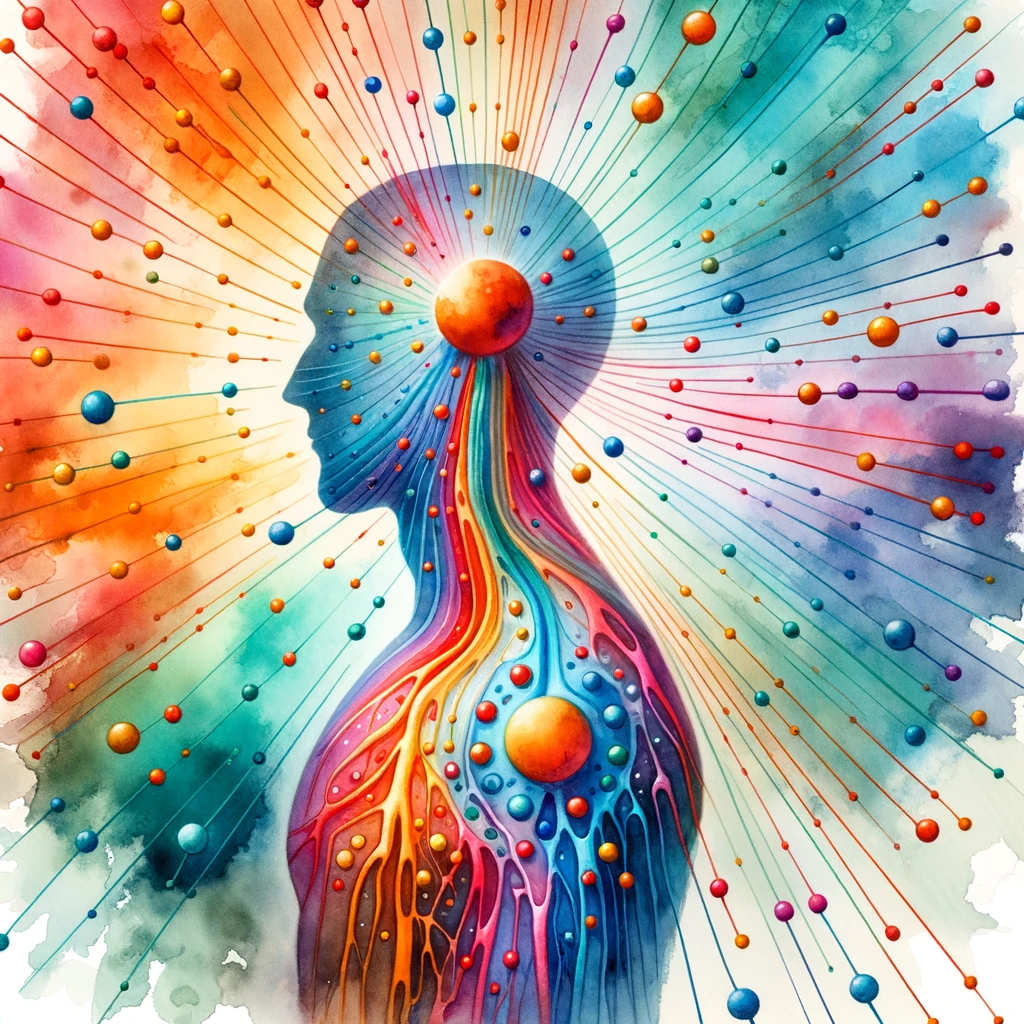This image is an abstract drawing of a human figure rendered in a pseudo-realistic silhouette, facing left. The figure, shown only from the head down to the torso, lacks any hair and features a clear profile of the nose and mouth. The silhouette is intricately constructed using watercolor splotches in various shades of orange, pink, blue, and purple that also create the striking background.

The head of the figure prominently features an orange ball positioned near the center of the skull, from which multicolored rays extend outward. These rays, resembling veins or threads, are adorned with multi-sized colored orbs that match the vibrant watercolor palette of the background, including shades of red, orange, blue, and purple. Another orange ball is situated on the shoulder, connected by similar multicolored rays. The overall composition presents a surreal blend of colors and abstract forms, creating a vivid, dynamic, and almost cosmic visual experience.